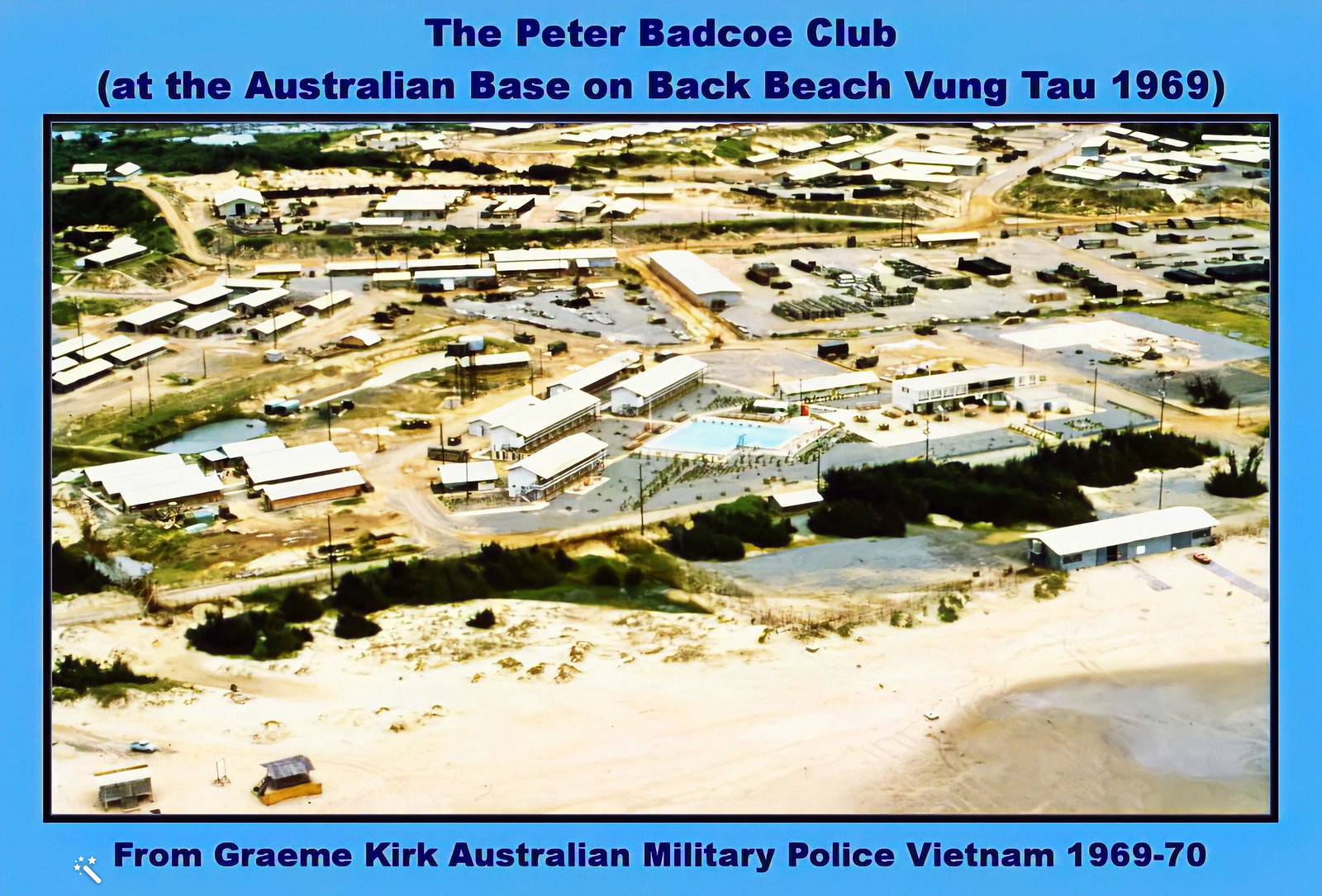The photograph, outlined by a blue frame, is titled "Peter Badko Club" with a subtitle in parentheses reading "at the Australian base on Back Beach, Vung Tau 1969." Additionally, the caption at the bottom credits "Graham Kirk, Australian Military Police, Vietnam 1969-1970." The image depicts a broad, tan and gray hued settlement or army base, comprised of long buildings, numerous roadways, and expansive parking areas. The scene includes details of military transportation, barely discernible due to the distance. In the foreground lies a vast, sandy, and wet area, possibly a beach, flanked by some scattered trees, shrubs, and bushes. The overall scene exhibits a predominantly bare, earthy expanse with minimal greenery.